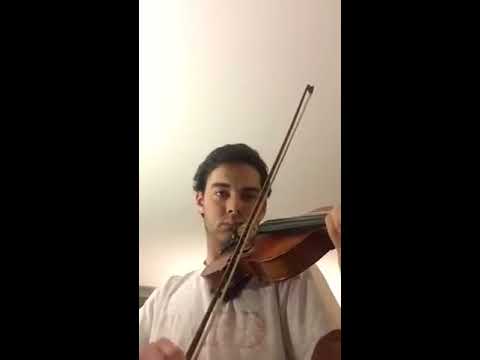This is a detailed indoor portrait-style photograph of a young man playing a violin, captured by a mobile phone. The man, who is wearing a white t-shirt with faded red lettering, has a serious expression on his face. He stands against a backdrop of a white ceiling and is bathed in partial light from an unseen source behind him. His dark, short, and slightly curly hair frames his face. He holds the violin on his left shoulder, gripping the neck with his left hand, while his right hand expertly maneuvers the bow across the strings. The camera, positioned at chest level, captures him from about the mid-torso upwards, with thick black bars on either side framing the image. The brown, wooden violin complements the simplicity of his attire and the intense focus in his eyes as he looks slightly down towards the camera.